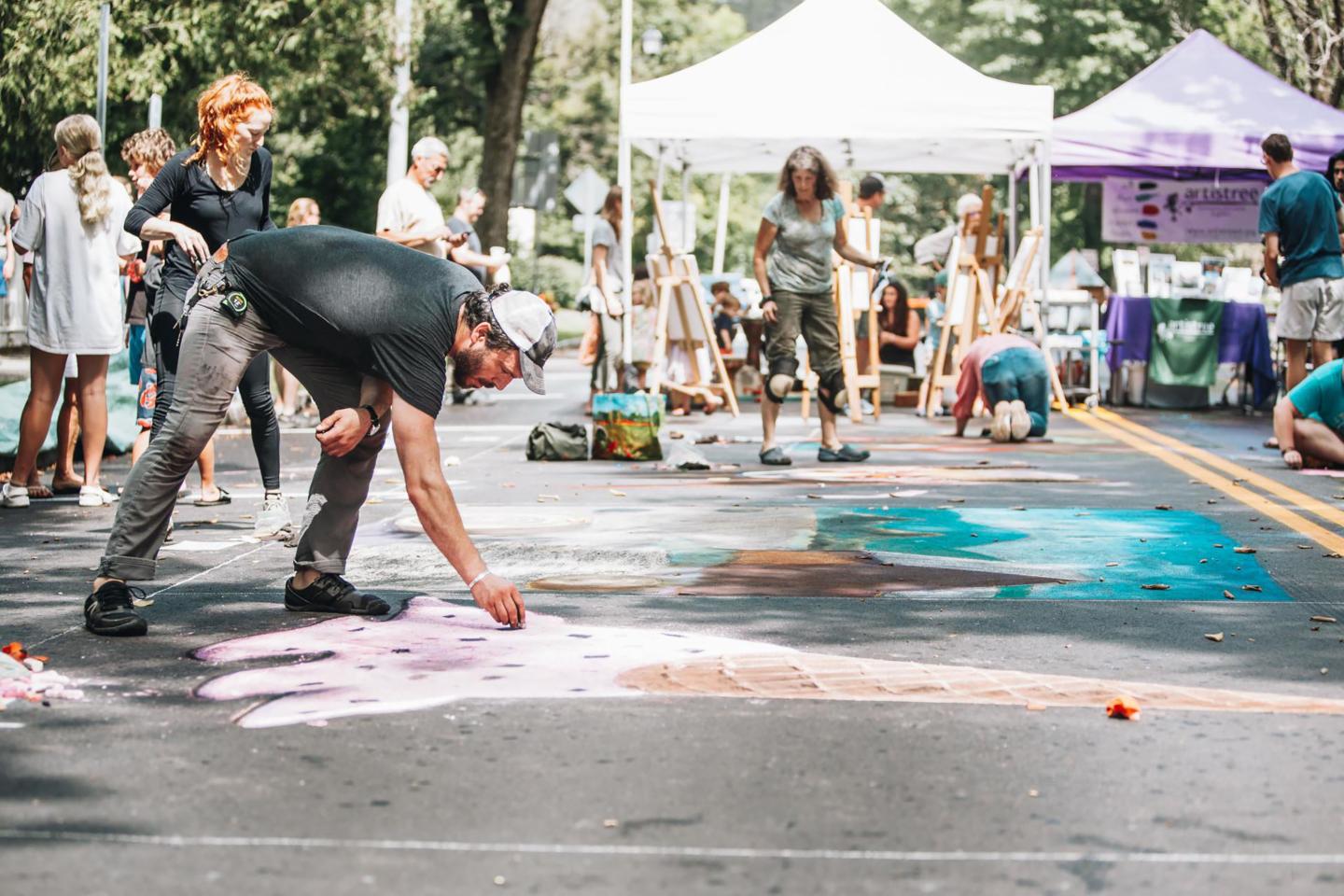In this vibrant outdoor photograph, we're at a bustling street art festival set against the backdrop of lush greenery and large trees. The scene is alive with activity and creativity, featuring colorful pop-up tents showcasing a variety of items for display or sale. The street is sectioned off with chalk lines, designating areas for artists to create their masterpieces directly on the pavement. In the foreground, a young man in a cap, black t-shirt, tennis shoes, and light black pants bends over a detailed chalk drawing of a fallen ice cream cone, his intense focus evident as he perfects the image. Nearby, a bright blue chalk drawing adds a splash of color. Two women watch him closely, appreciating his artistic efforts, while other festival-goers of all ages, from children to the elderly, explore the concessions, easels, and other art setups around them. Little wooden frames for canvases stand ready for more artistic endeavors, amplifying the creative atmosphere of this lively street art celebration.